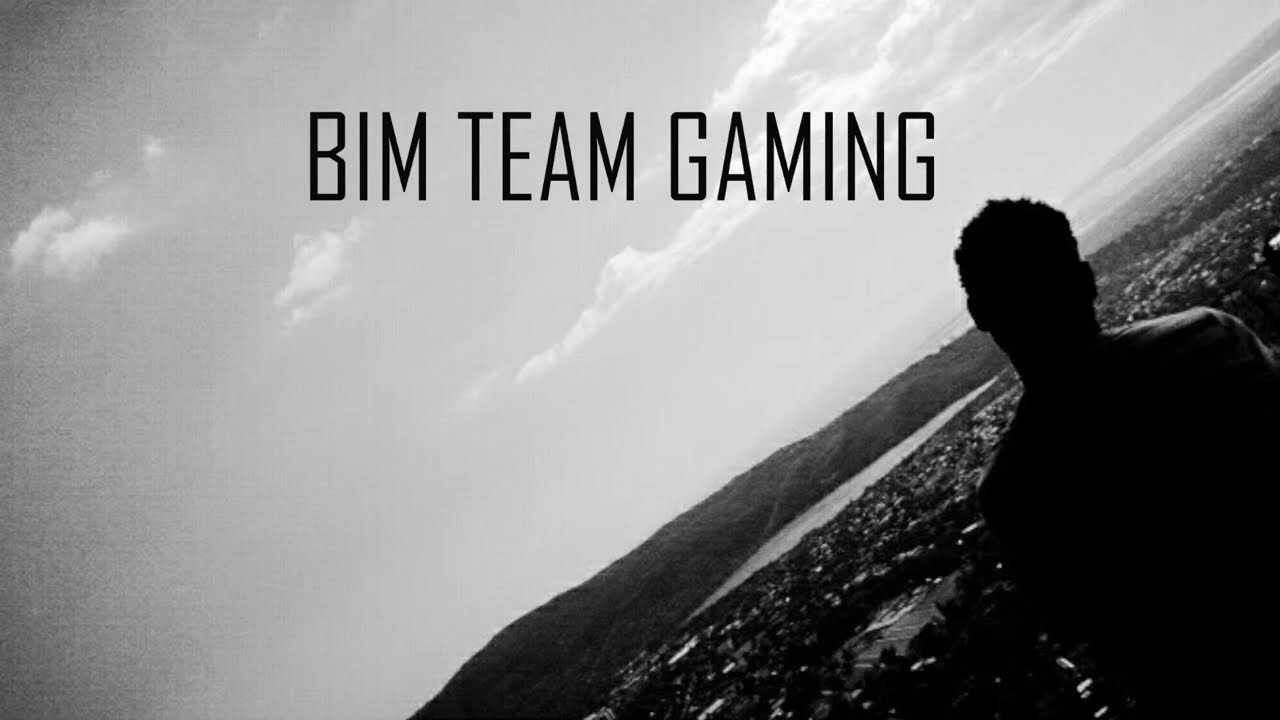The photograph, presented in black and white, is tilted slightly, creating a sense of dynamic movement. The vantage point begins around the 10-30 positions in the upper left corner in a landscape perspective. The top two-thirds of the image features a partly cloudy sky, hinting it's daytime due to the visible clouds. Below the sky, a hill or small mountain range covered with trees descends into a small body of water, potentially a lake. Further down, the subtle outlines of a cityscape emerge, suggesting subdivisions and commercial buildings, though the poor lighting blurs most details into dark masses.

Dominating the lower right corner is the silhouette of a man, standing and looking out over the city. His back is likely facing the viewer, inferred from the outline of his shoulders, though it remains ambiguous. Across the top center of the image, in thin capital letters, aligned neatly, reads "BIM Team Gaming," adding a distinct layer of text to the visual.